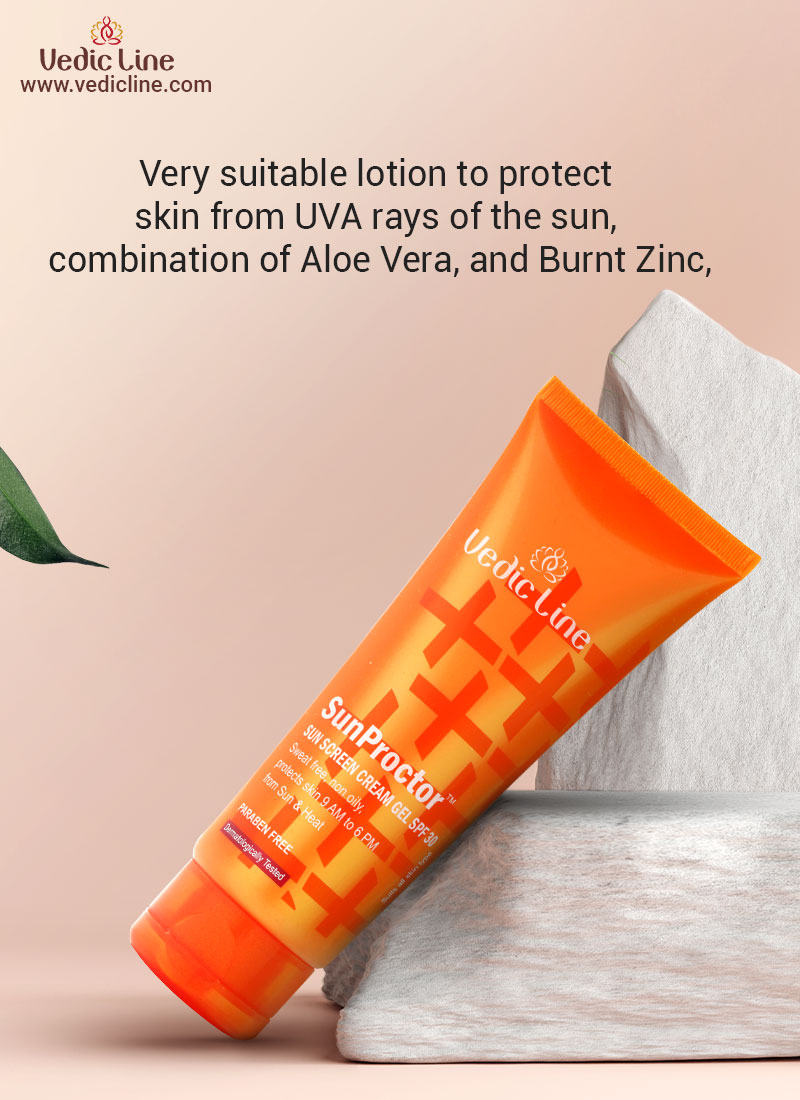This is an advertisement for Vedic Line's Sun Protector sunscreen cream gel with SPF 30. The ad features an orange bottle adorned with orange pluses, angled against white, striated rocks amidst a light pink background. The top left corner displays the brand name and website: Vedic Line (www.vedicline.com). Centered at the top, black text reads, "Very suitable lotion to protect skin from UVA rays of the Sun. Combination of aloe vera and burnt zinc." To the middle left of the image, a green leaf protrudes subtly. Additional text on the bottle highlights that it is dermatologically tested.